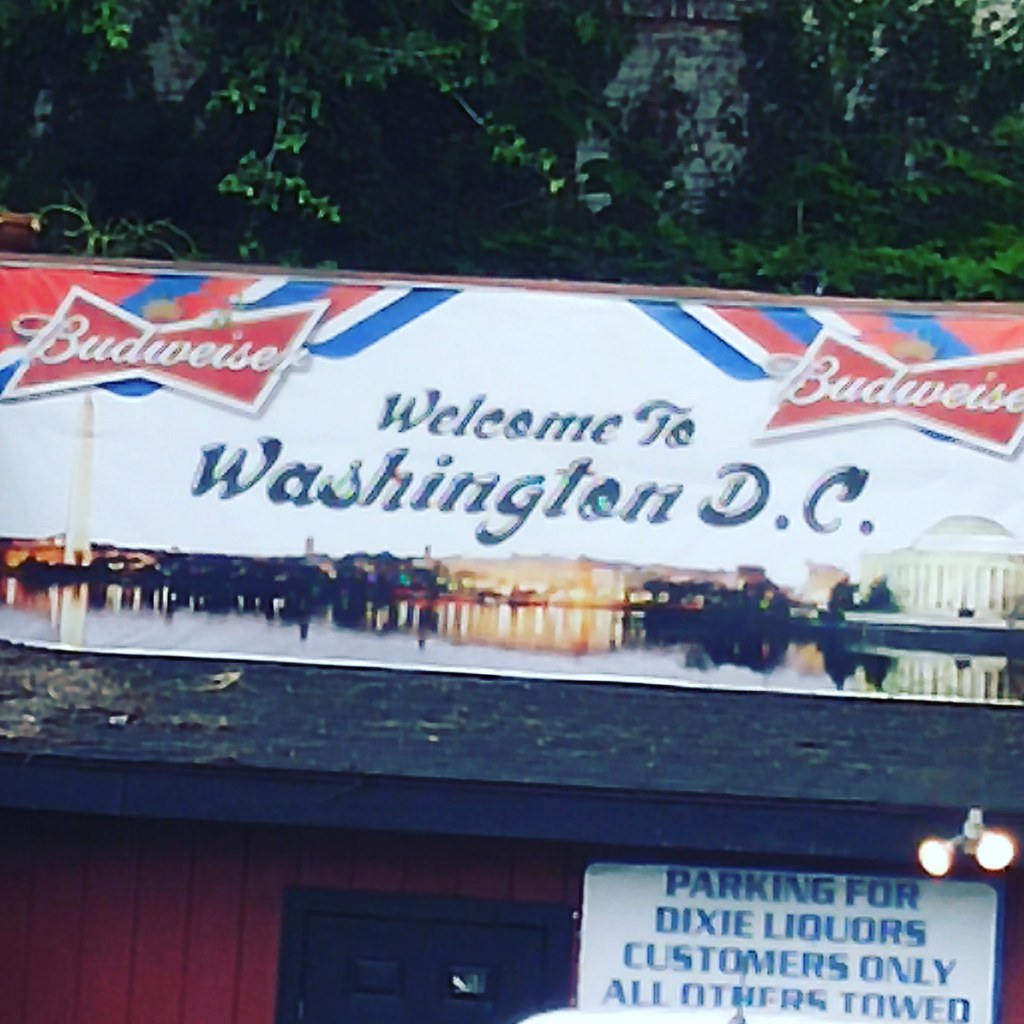This photograph captures the vibrant facade of a building, likely a bar named "Dixie Liquors," situated in an urban setting. Prominently displayed is a white sign in the lower right corner that reads, "Parking for Dixie Liquors customers only, all others towed," in dark blue lettering. A large banner or sign dedicated to Budweiser dominates the upper portion of the building. The sign features the text "Welcome to Washington DC" in the center, also in dark blue letters, set against a white background. Flanking this text are two distinctive Budweiser logos, each resembling two triangles joined at the tips, with "Budweiser" elegantly scripted in white against a red background. Enhanced by red, white, and blue striped flags, these logos add to the establishment's patriotic decor. In the background, a house, trees, and bushes provide a glimpse into the surrounding neighborhood, adding depth and context to the setting.